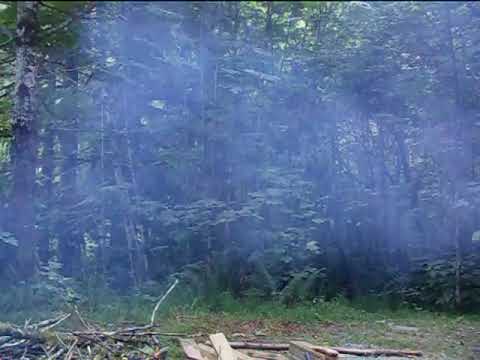The image depicts a densely wooded forest with a tree line that rises with fairly skinny trunks, showing various kinds of dense foliage. In the background, the trees are shrouded in a layer of smoke, making visibility difficult and giving the scene a blurry and pixelated appearance, reminiscent of a low-resolution video frame. In the foreground, there's a flat, sparsely grass-covered clearing littered with wood debris, including a small pile of branches and twigs in the bottom left. To the right of this pile, treated 2x4 wooden planks are scattered, suggesting they may be part of a structure or a makeshift ramp. The pervasive smoke hints at possible burning activities or another source of heat, although the source itself is not visible in the image.